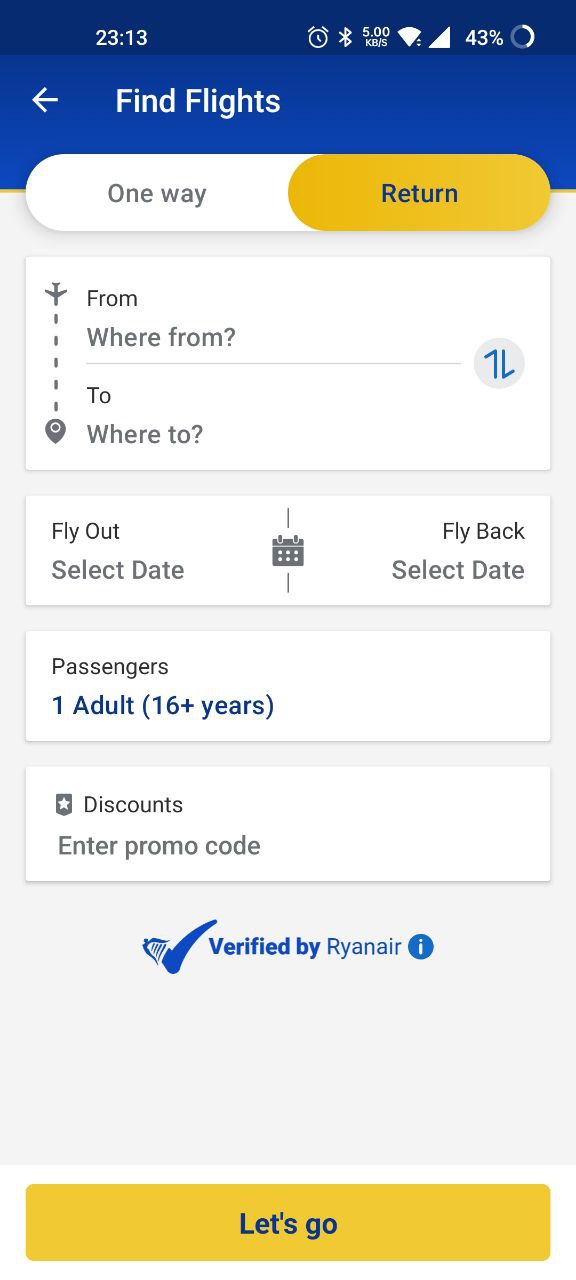The image appears to be a screenshot from a mobile device, taken at 11:13 PM, displaying a flight search interface, possibly from a website or an app. At the top of the screen, next to the notification icons, the page prominently reads, "Find Flights." Users can choose between "One Way" or "Return" flight options. Below that, there are fields labeled "Where From" and "To Where," allowing users to input departure and destination cities. 

Further down, users can "Select Date" for both the "Fly Out" and "Fly Back" options. Other options include setting the number of "Passengers," which currently reads "One Adult" (defined as individuals 16 years and older). There is also a section for "Discounts," where users can "Enter Promo Code." The platform is verified by Ryanair, indicated by a small blue icon with an 'i' for more information. 

Towards the bottom of the image, there's a yellow clickable box labeled "Let's Go." The phone's status bar shows that Bluetooth is enabled, an alarm clock is set, Wi-Fi is connected with a good signal, and the battery level stands at 43%.